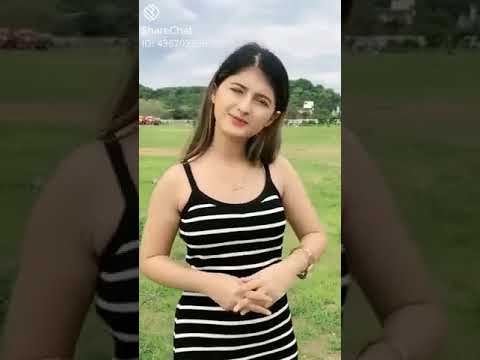The image features a young woman of Asian appearance, likely in her early 20s. She has long, dark brown hair that falls just past her shoulders and is pulled behind her ears. She stands outside in a grassy field, with a hill adorned with trees and vegetation visible in the background. The day appears overcast. She is wearing a sleeveless, black and white striped spaghetti strap dress and has a fine gold chain necklace around her neck, complemented by a gold watch and bracelet on her left wrist. Her hands are gently clasped in front of her torso, and she has an odd expression on her face, possibly squinting due to the sun. This image is likely a screen capture from a video stream, indicated by its low to medium quality. The overall image is zoomed out, with a zoomed-in splice of the same image with a dark filter overlay. Additionally, there is text in white lettering, perhaps a logo or name with an ID number, in the top left corner, although it's too blurry to decipher. The image size is approximately 6 inches wide by 5 inches tall.